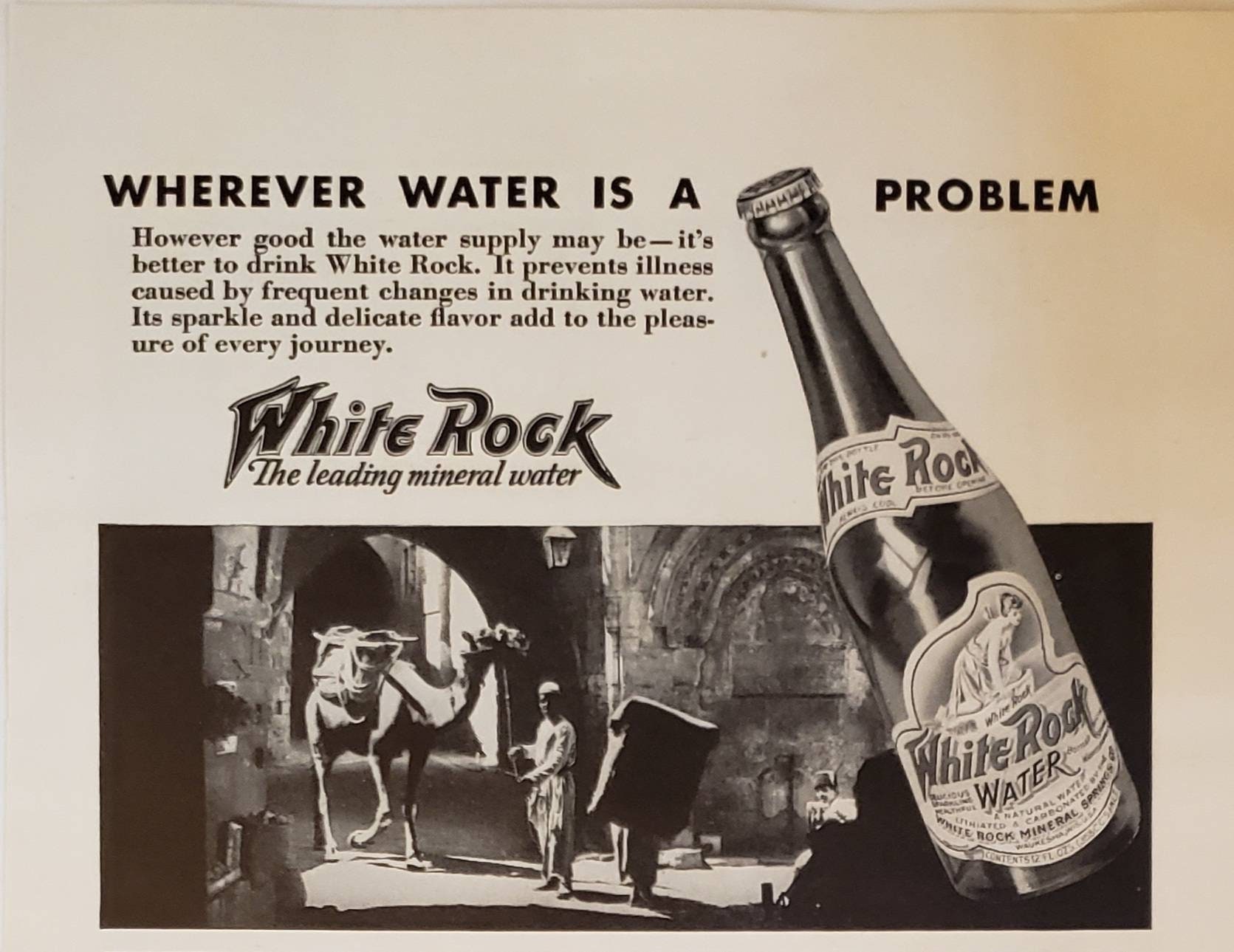This vintage black-and-white advertisement for White Rock mineral water appears to be from an old newspaper or magazine. The ad prominently features the tagline, "Wherever water is a problem," followed by the message, "However good the water supply may be, it's better to drink White Rock. It prevents illness caused by frequent changes in drinking water. Its sparkle and delicate flavor add to the pleasure of every journey." The centerpiece of the advert is an image of a White Rock mineral water bottle, described as the leading mineral water. To the right of the text and below the bottle, there is a striking black-and-white photograph of a man standing next to a camel along a stone pathway. The camel is laden with goods, indicating it is used for hard labor, while stone arches frame the background, adding to the nostalgic and historic feel of the advertisement.